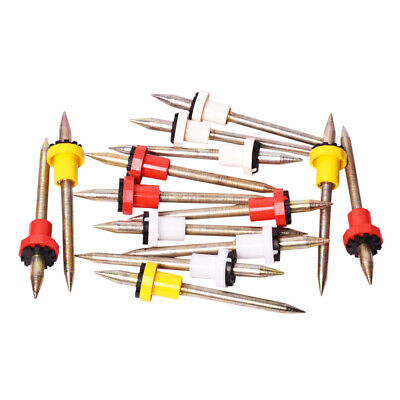In the image, there is a collection of double-ended, spear-like nails, displayed on a completely white background. Each nail has a sharp point on both ends and features a plastic cap situated just below one of the points. These caps come in red, yellow, and white and are adorned with small sections of black rubber-like material, which appears to be slit-proof. Scattered across the background, the nails are laid out in a somewhat haphazard fashion, with some appearing in the foreground and others slightly further back. These items, numbering around a dozen, look like specialized tools, although their exact purpose is unclear.